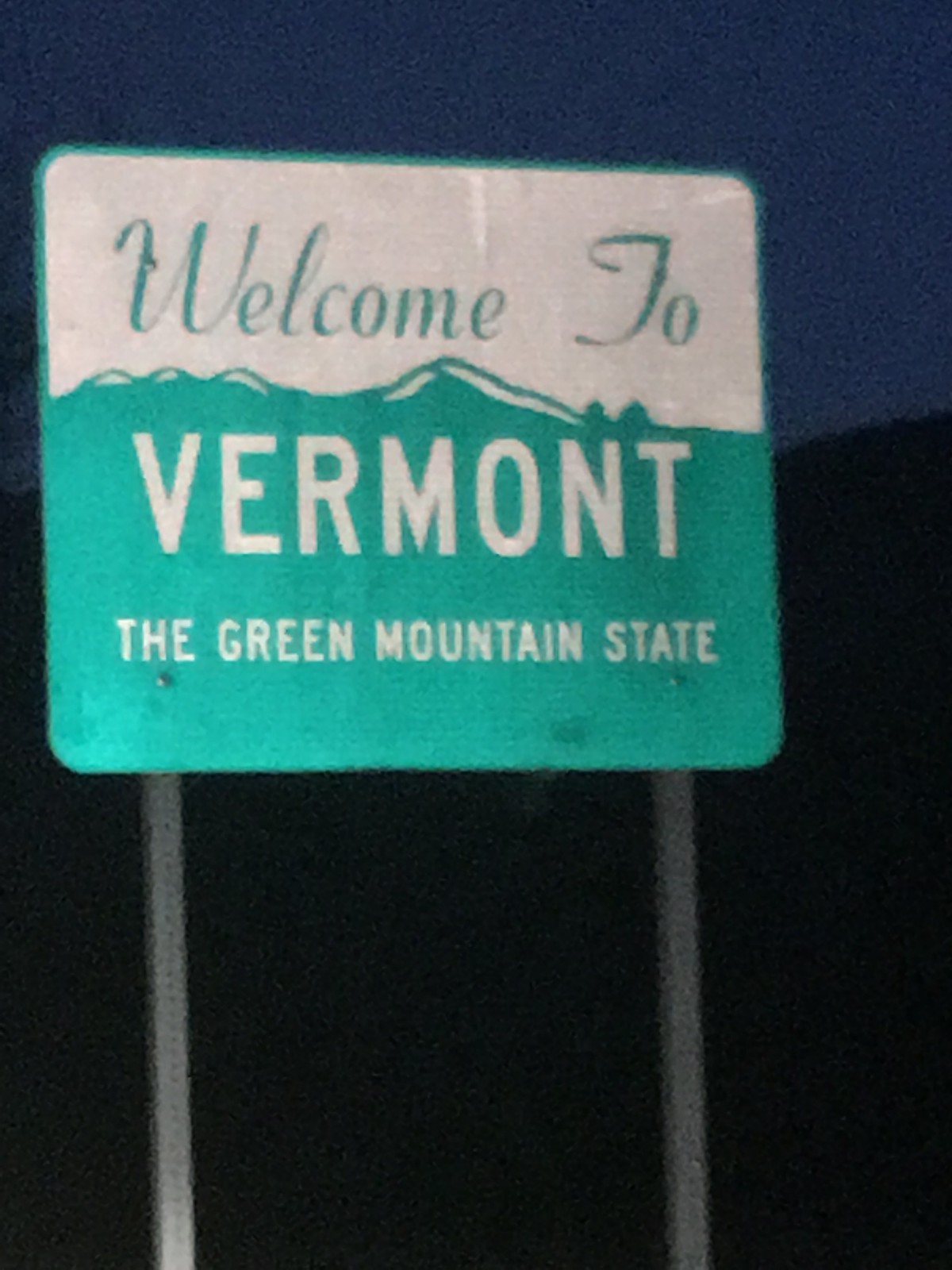Captured in the quiet hours of either nighttime or the early morning before sunrise, this image focuses on an outdoor roadside sign welcoming travelers to Vermont. The sign prominently features a backdrop of dark green, over which the phrase "Welcome to Vermont" is highlighted in a light green color. The bottom portion of the sign is distinguishable by its lighter green shade, while the upper section is a crisp white. "Vermont - The Green Mountain State" is clearly inscribed in white letters, making a striking contrast against the green base. The zoomed-in shot meticulously details the sign's colors and text, encapsulating a sense of serene anticipation as one enters the picturesque state of Vermont.